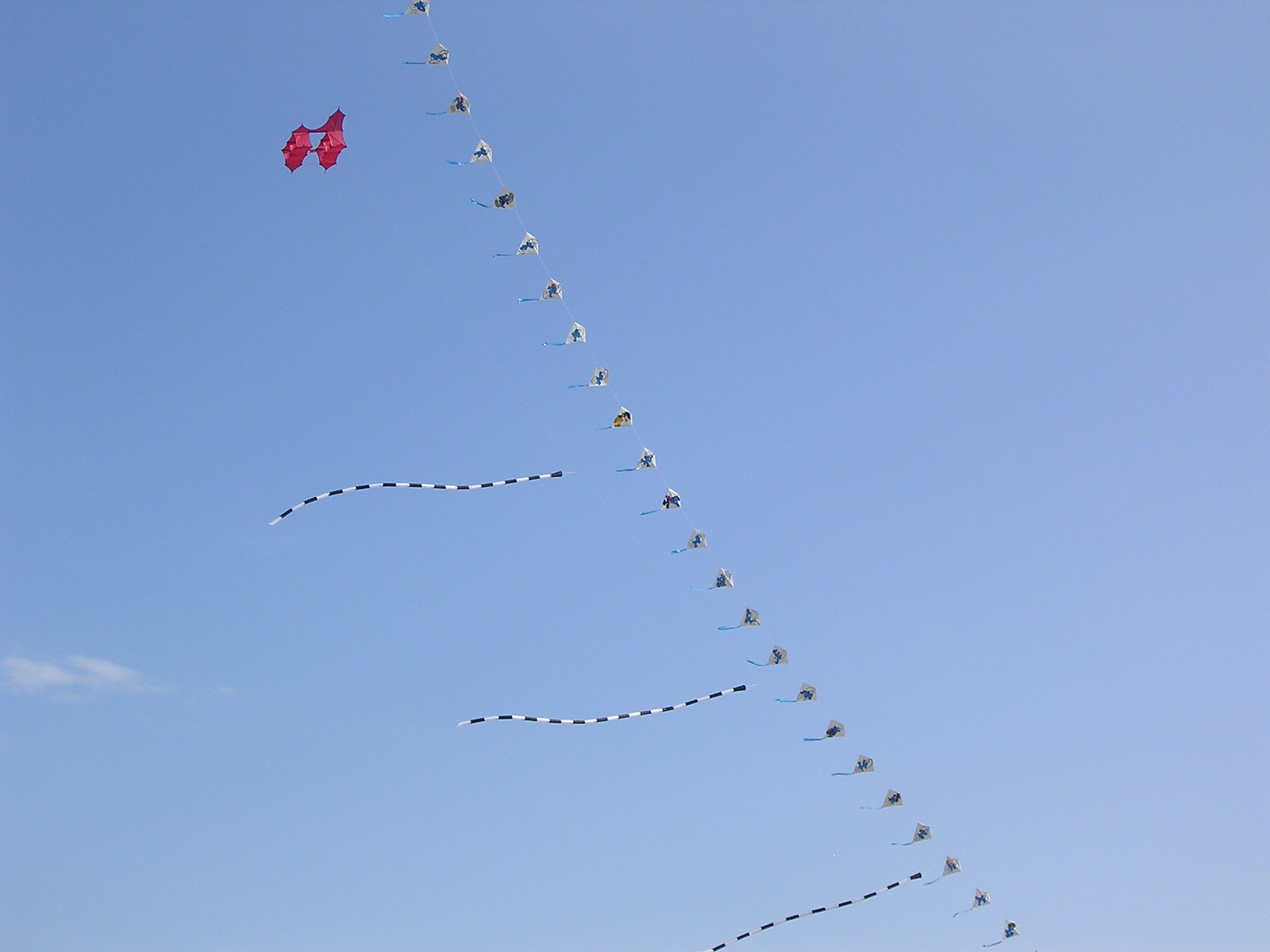The photograph captures a vibrant, clear day with a bright blue sky punctuated by a single small cloud in the lower left corner. Dominating the image is an impressive string of at least 24 interconnected kites stretching vertically upwards. The primary kites along the string are traditional diamond-shaped, adorned with blue tails. Every few kites, there are offshoots featuring long, black and white kites hanging horizontally. These distinctive horizontal kites appear three times along the string. Near the top of this vertical arrangement is a striking red, two-piece kite design, which adds a three-dimensional effect to the scene. Additionally, another element in the image is a pink detail hanging from one of the kites, enhancing the overall colorful and dynamic composition.